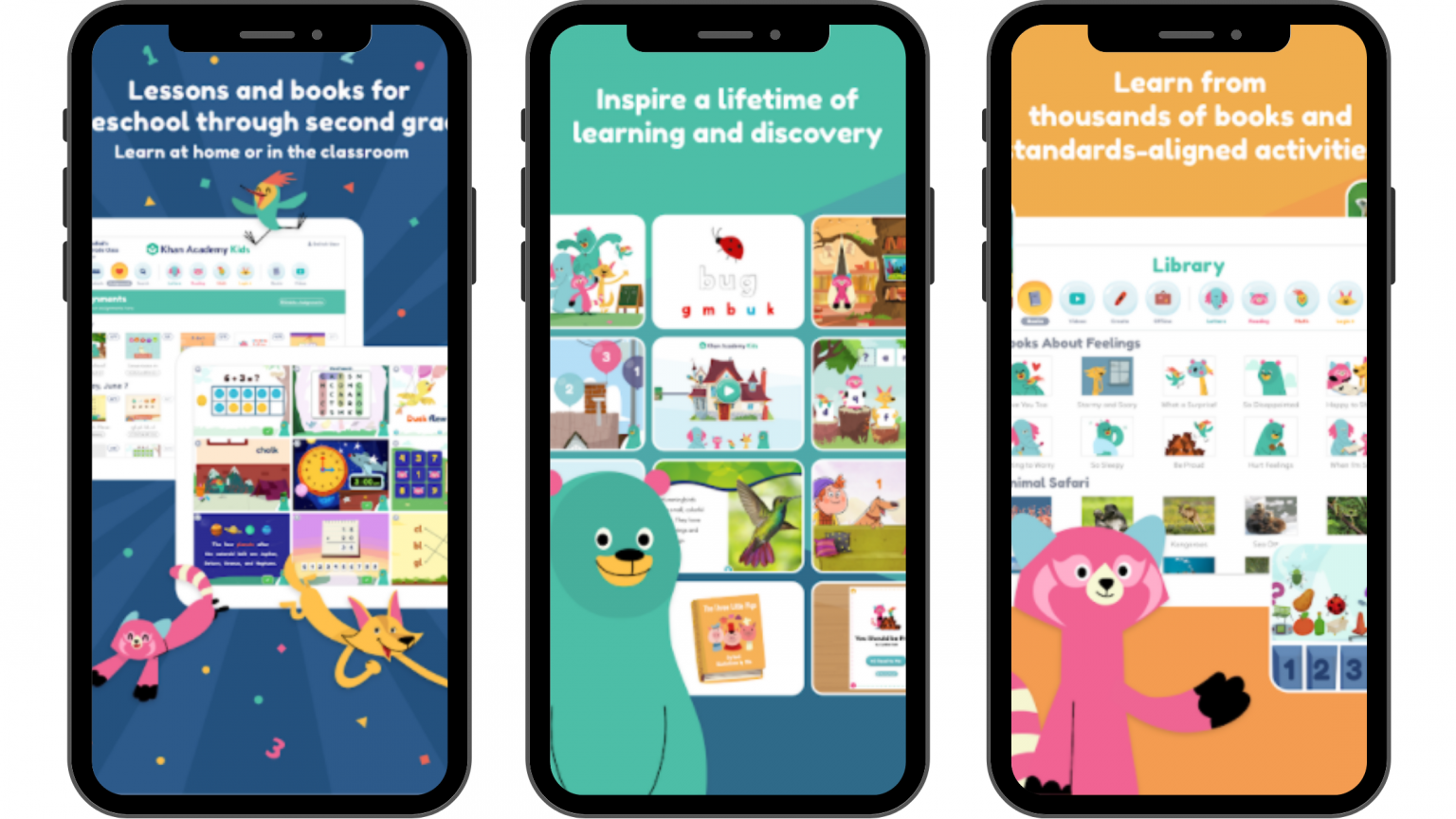Here are three detailed captions for the given screenshots:

1. **Screenshot 1:** "The first screenshot showcases a collection of educational lessons and books for e-school, targeting students from kindergarten through second grade. The interface features a cheerful bird with red hair perched at the top against a blue background, enhanced with celebratory confetti. Various webpages from Khan Academy for Kids are displayed, including simple children's puzzles. On the right side, a dynamic yellow wolf with a prominent streak down its forehead is diving forward, while a uniquely colored red panda with pink fur and white-striped tail, detailed with blue ears, adds an element of fun and engagement."

2. **Screenshot 2:** "The second screenshot shows an inspiring message: 'Inspire a lifetime of learning and discovery,' accompanied by a whimsical blue-teal bear with a slightly darker face and pink ears. The screen highlights educational puzzles designed for young children, offering a range of activities such as scrambling puzzles, reading exercises, and foundational math problems, all targeted at pre-kindergarten learners."

3. **Screenshot 3:** "The third screenshot features vibrant orange bars at the top and bottom with the aforementioned uniquely colored red panda, boasting light pink markings on its face, blue ears, a pink body, and white stripes. It emphasizes access to a vast array of books and standards-aligned activities. There’s a library option showcasing subjects like animal identification, math, writing, and general kindergarten or preschool activities, aimed at fostering early educational development."